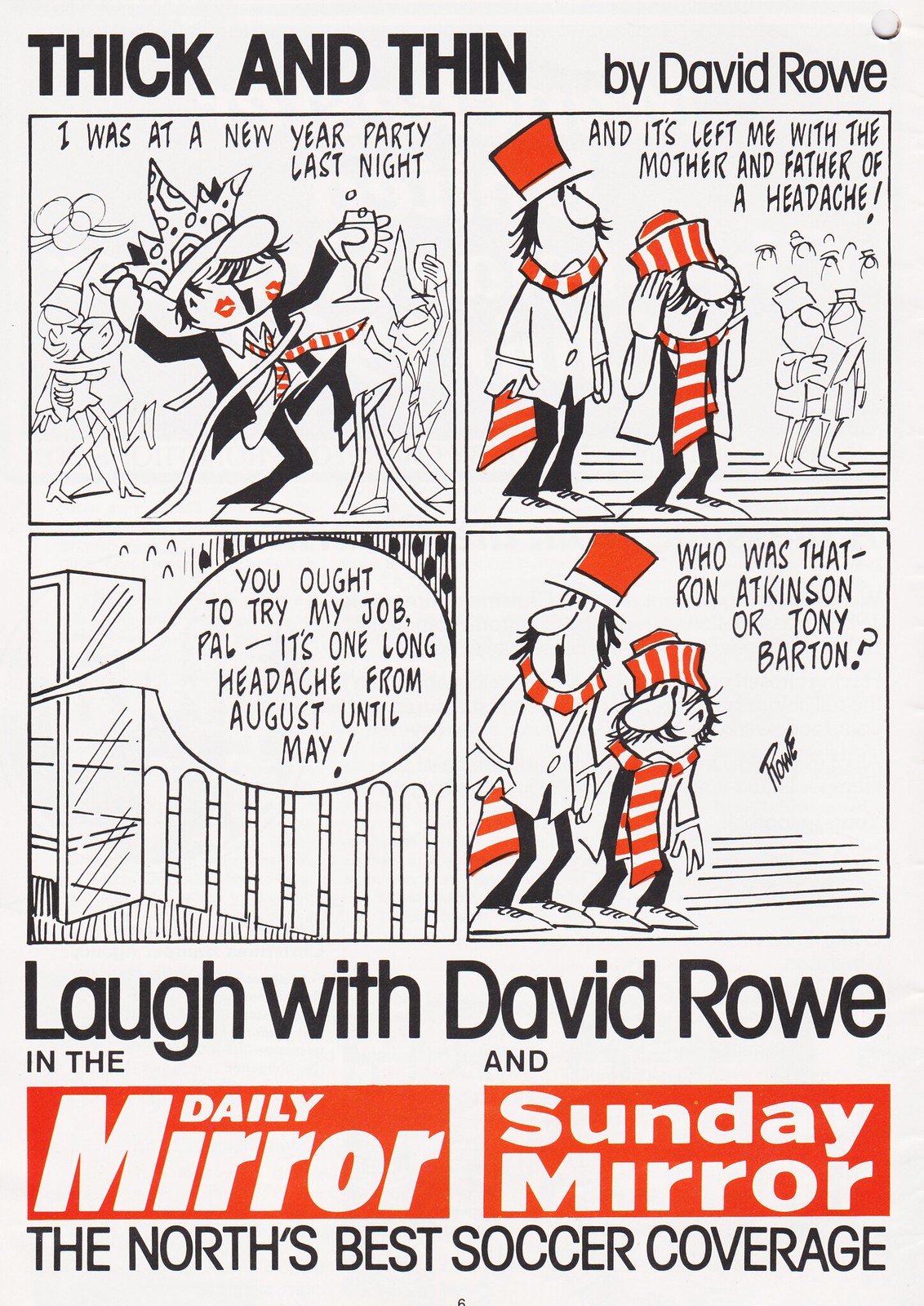The comic strip, titled *Thick and Thin by David Rowe*, prominently features black, white, and red colors. The comic begins with a man in a black suit, white shirt, and a red-and-white striped tie, wearing a crown and holding a glass, with two lipstick marks on his cheeks. He says, “I was at a New Year’s party last night.” Next to him, the panel caption continues, “It’s left me with the mother and father of a headache.” The adjacent panel reveals the same man now in a white jacket alongside another character also in a white jacket, black pants, and an orange-and-white scarf and hat. The text bubble says, “You ought to try my job, pal. It’s one long headache from August until May.” In the final panel, the two characters stare at one another, with a dialogue that reads, “Who was that, Ron Atkinson or Tony Barton?” Below the comic, there's a footer that reads, “Laugh with David Rowe in the Daily Mirror and Sunday Mirror, the North’s best soccer coverage.”